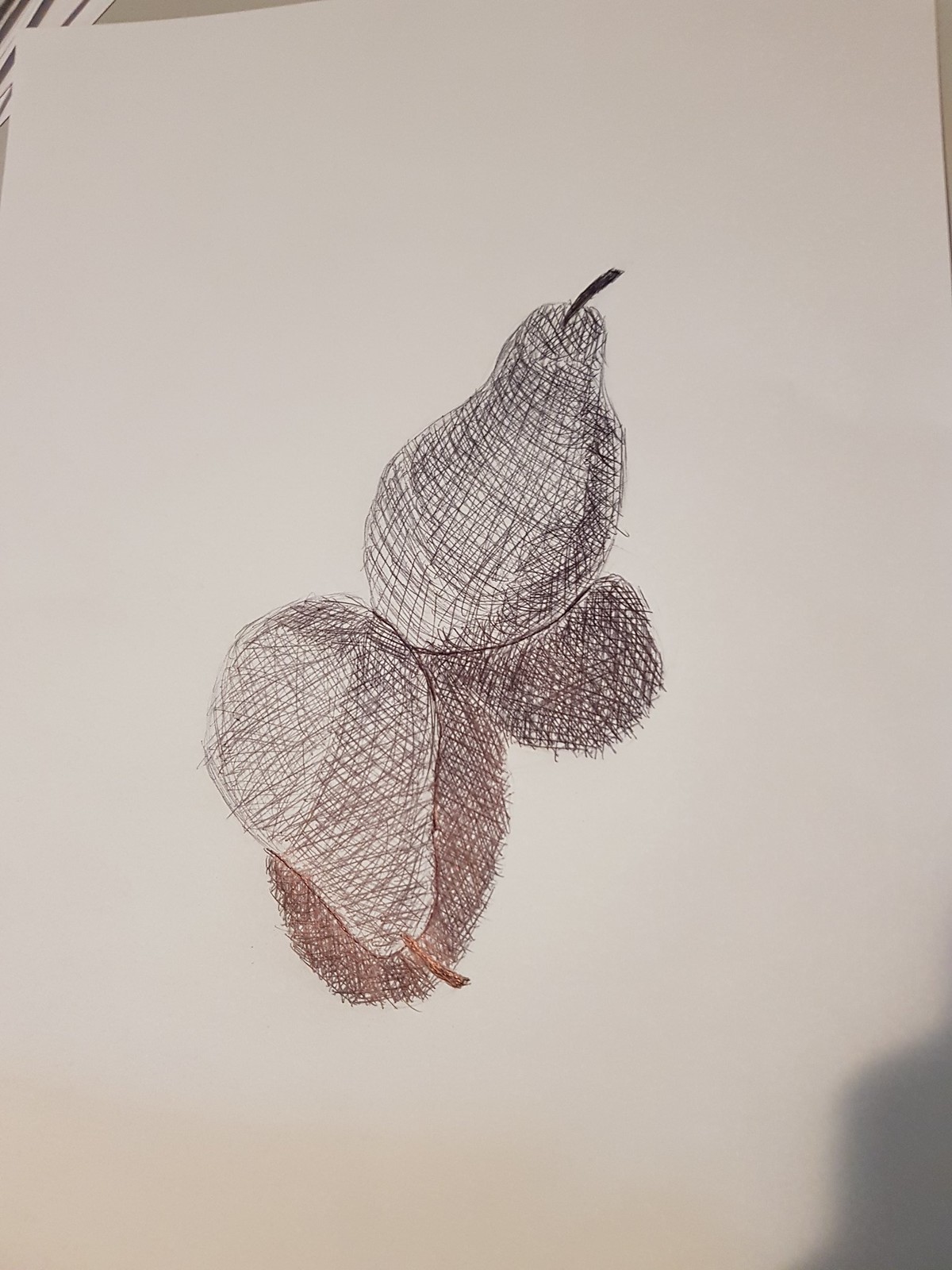The image is a vertical photograph of a hand-drawn still life featuring two pears on an off-white sheet of paper. Both pears are rendered with intricate crosshatch shading, likely done in pen or pencil. The upright pear, positioned with its stem at the one o'clock direction, has a darker stem, while the pear lying down, pointing towards five o'clock, has a lighter, brown stem. Shadows are meticulously sketched, primarily on the right side and under the reclining pear. The background reveals part of a dark cream table and a second sheet of paper with black and white stripes underneath the main paper, visible in the upper left-hand corner. The bottom right-hand corner of the image also includes a shadow, enhancing the sense of depth in this detailed still life.